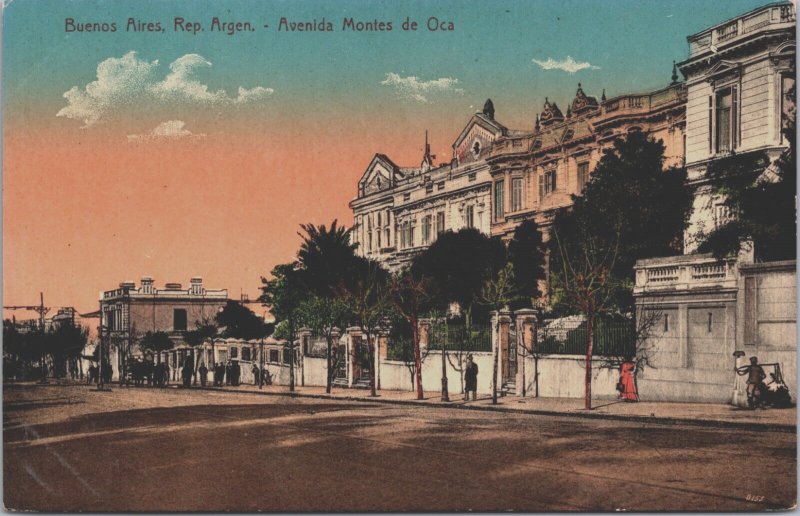This vintage, hand-colored postcard depicts a picturesque street scene in Buenos Aires, labeled at the top with "Buenos Aires, Rep. Arjun, Avenida Montes de Oca" in a distinctive reddish-orange font. The sky transitions from a tranquil blue at the top to an orangey-peach hue near the horizon, adorned with wispy white clouds. Dominating the right side of the image, there is an elaborate, large white building characterized by intricate architectural details and topped with decorative railings. This building is part of a row of three sizeable structures, each varying slightly in color from bone white to a subtle reddish tint, all standing three stories high. In front of these buildings runs a substantial stone wall, with green trees interspersed between the wall and the edifices. The broad, brownish pavement below is speckled with the shadows of pedestrians. These individuals, dressed in vintage attire—women in elegant, long dresses and men in suits—wander along the street, giving a glimpse into a bygone era. As the warm hues of sunset illuminate the scene, it evokes a serene, nostalgic atmosphere, capturing a moment of calm in the bustling city.